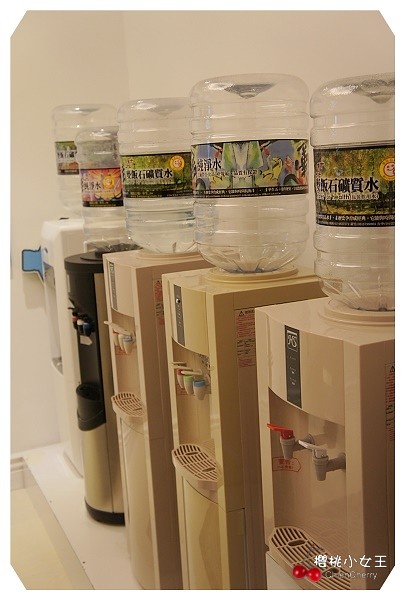This colour photograph depicts a row of five water coolers, commonly found in office environments, aligned from the foreground on the right to the background on the left. Each water cooler features slight design variations, with differences in the number of taps – some having two while others have three. The nearest cooler in the foreground has a mix of tap colours: one red-topped on the left, a white-topped on the right, and the tap bodies are grey. Below the taps, there is a mesh tray designed to collect spillages.

All coolers are topped with large, inverted plastic water bottles, adorned with vibrant, heavily patterned labels that have black Japanese characters. The bottles also show round ridges around their circumference. The coolers vary in colour and material: the closest one is white, another is black and metallic, and the rest range in shades of tan and beige. The floor is beige and there appears to be a beige bar running under the coolers, which could be part of the room’s structure. 

The image has a yellowish tinge, suggesting poor indoor lighting or a filter effect. Additional elements include a blue square shape on the wall to the far left and Chinese characters in white found in the lower right-hand corner of the photograph, alongside some barely legible English text.